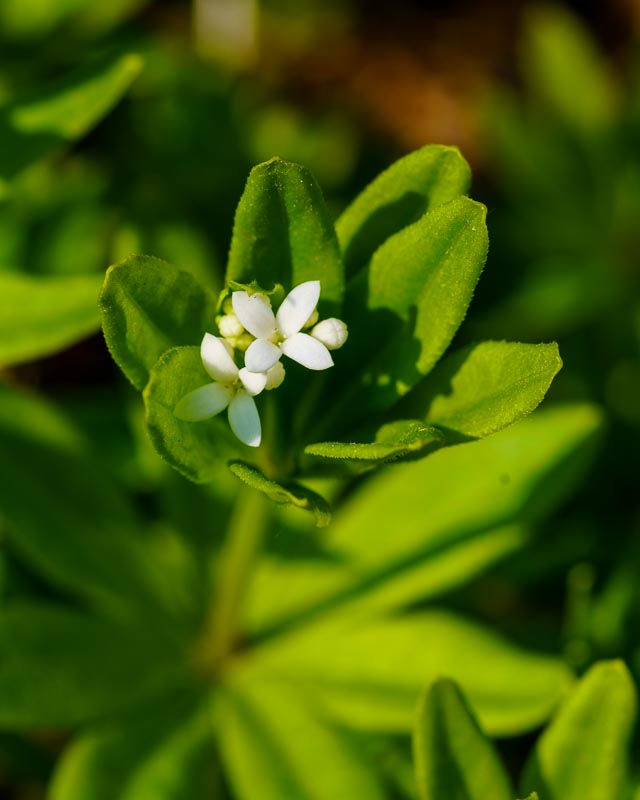This vertical, rectangular photograph showcases a tiny white flower nestled protectively within its much larger green leaves. The leaves, arranged in a cup-like formation, surround the flower, which is reminiscent of an edelweiss flower, featuring four delicate petals and small yellow centers. Positioned at the focal point in the center of the image, the flower, and its encompassing leaves stand out crisply against a blurred green backdrop, emphasizing the plant's intricate details. The perspective gives the impression of looking straight down at the plant, capturing the rich, vibrant green hues and the detailed textures of the leaves, which vary from light to dark green. Surrounding the central focus, other similar but out-of-focus plants create a soft, green backdrop, adding to the modern and visually striking composition of the photograph.